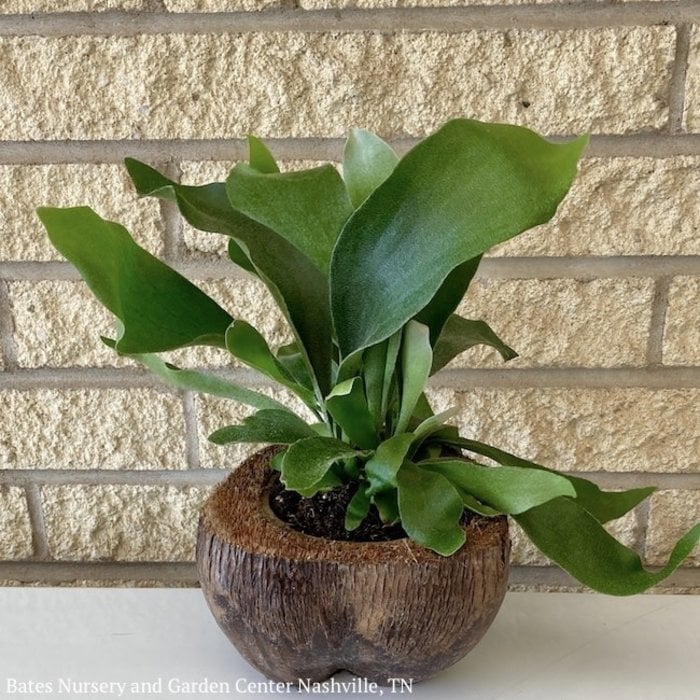This square photograph captures a potted plant set against a backdrop of cream-colored brickwork with light gray grout. The plant sits in a medium-sized, dark brown pot that resembles the texture and shape of a coconut shell. The pot, containing dark brown dirt, hosts a lush plant with a combination of short and long, broad, vibrant green leaves—some extending gracefully downward and curling upwards. The plant is placed on what appears to be a light gray or white surface, potentially a concrete shelf that blends with the brick wall behind it. Notably, the lower left corner of the image features white text that reads, "Bates Nursery and Garden Center, Nashville, Tennessee," suggesting it is an advertisement for the nursery. The photograph is devoid of any people or animals, focusing entirely on the botanical display.